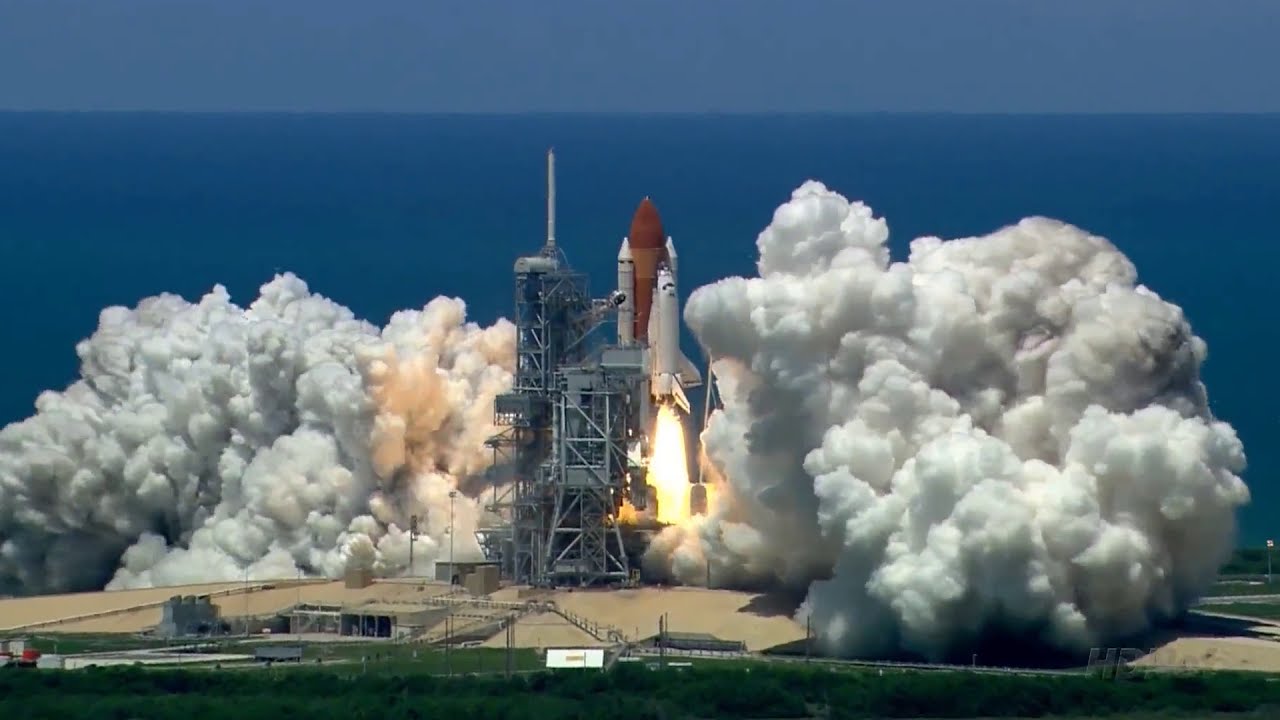In this realistic photograph, a rocket launch is captured in vivid detail, moments after liftoff. The rocket, prominently positioned in the center of the image, comprises a white space shuttle with black windows, mounted on three large boosters—one red central rocket flanked by two white rockets. Brilliant flames burst from the base, casting an intense glow and creating immense billows of smoke on either side, almost reaching the height of the nearby scaffolding structure made of gray metal.

The scene is set against a dramatic background: a dark blue sky transitioning to a lighter blue line above the horizon, meeting the ocean below. A distinct straight line separates the dark and light blue portions of the sky. The launch site sits on brown cement ground, behind which lies a metal fence topped with barbed wire. Beyond the fence, green bushes and a line of buildings are visible. The photo, likely taken from a high vantage point, also reveals patches of grass at the bottom, enhancing the composition with a touch of nature amidst the advanced technology of space exploration.